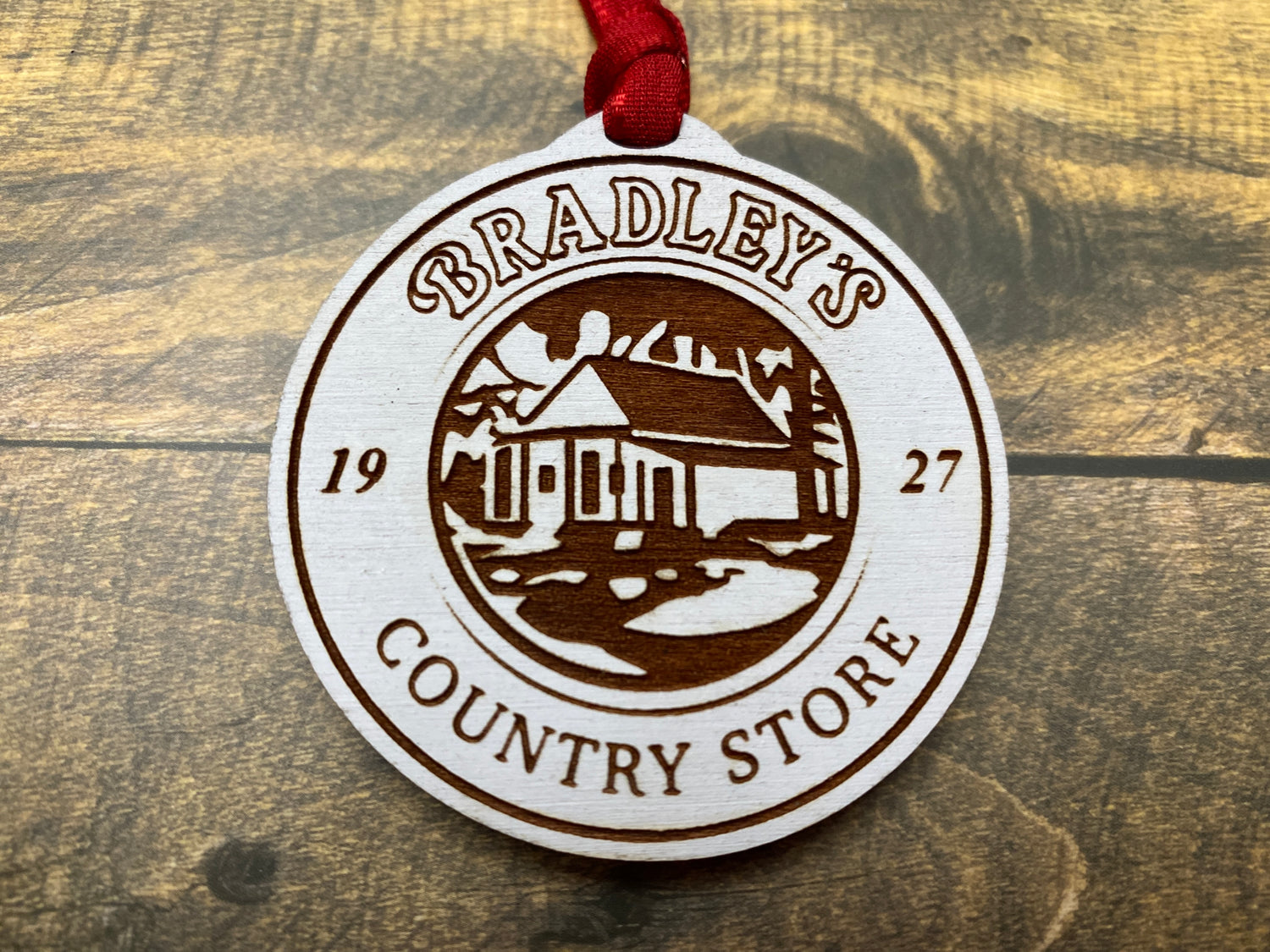The image depicts a circular wooden emblem resting on a dark wooden table with prominent grain patterns. The emblem itself is painted primarily white and bordered by a dark red circular outline. At the top, it features the text "Bradley's" in a red-outlined font, while the numbers "1927" appear on both the left and right sides. Bold red text at the bottom reads "Country Store." Central to the emblem is an outline of a quaint cottage, complete with visible features such as a doorway, a couple of windows, and surrounding trees. A red lanyard is tied to the top of the emblem, looping through a hole, further accentuating its rustic design.